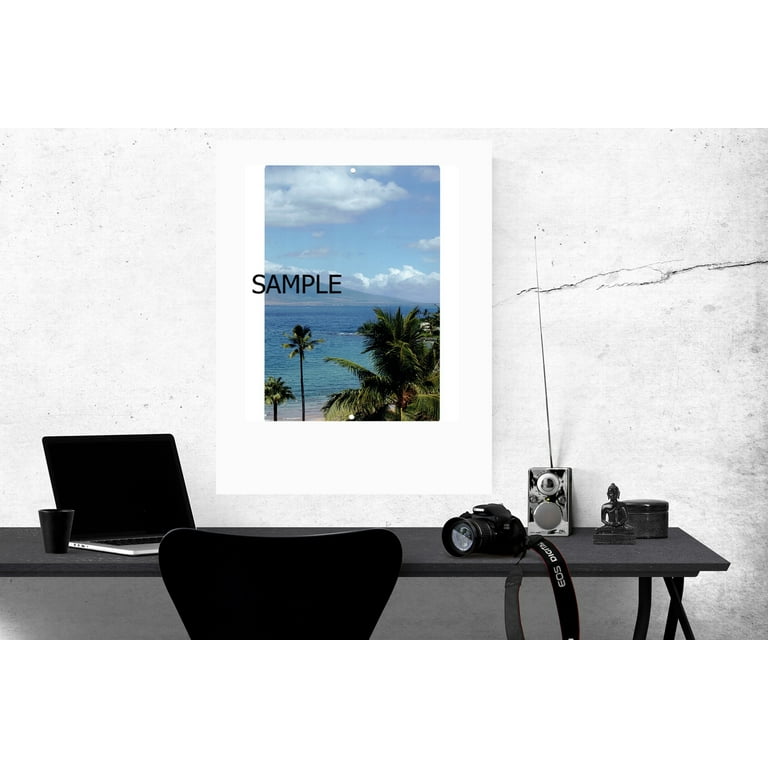A detailed photograph of a sparse black desk set against a light gray wall features an organized office-like setting. Central to the composition is a sleek, black desk with thin legs, supporting a laptop with a black screen and a visible silver keyboard partially obscured by the black square roll-top chair placed at the desk. To the left, a small glass, resembling a larger shot glass, sits nearby. On the right side of the desk, a professional 35mm camera with a strap draped over the table stands next to a black mug. Adjacent to the camera, there is a device with an antenna, likely a radio, coupled with a small Buddha statue in a lotus position. A round box with a lid and another small trinket complete the desk ensemble. Above this setup, a vibrant beach scene poster depicting a tropical vista with palm trees, clear ocean water, and a sky with fluffy white clouds adds a splash of color to the otherwise monochromatic scene. The word "SAMPLE" is printed across the sky area of the poster, emphasizing its illustrative purpose. The room's background, featuring gray walls, provides a calm and focused ambiance, making it an ideal space for tasks like photography editing or office work.